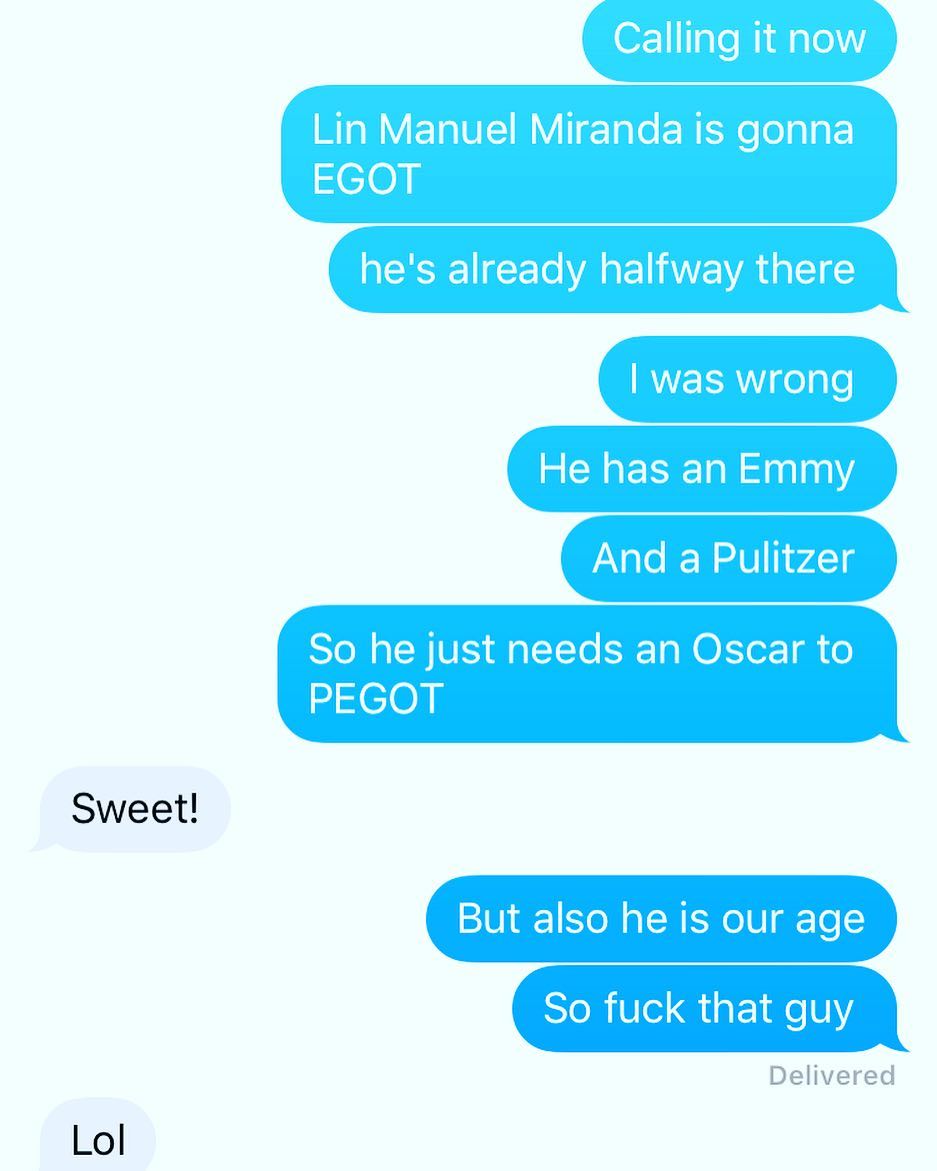The image is a screenshot of a text message conversation, displaying nine consecutive messages from one person on the right side of the screen and two replies from another person on the left. The initial sender's messages, shown in blue bubbles with white text, start with "Calling it now," followed by "Lin-Manuel Miranda is going to EGOT," "He's already halfway there," "I was wrong," "He has an Emmy," "And a Pulitzer," and then "So he just needs an Oscar to PEGOT." After this string of messages, the comment "sweet!" is seen in a white bubble with black text on the left. The original sender continues with "But also he is our age," and "So fuck that guy," with the last of their messages marked as delivered in gray text beneath it. The conversation ends with a final response from the other person on the left, saying "LOL." The text is large and clear, typical of a smartphone chat interface.